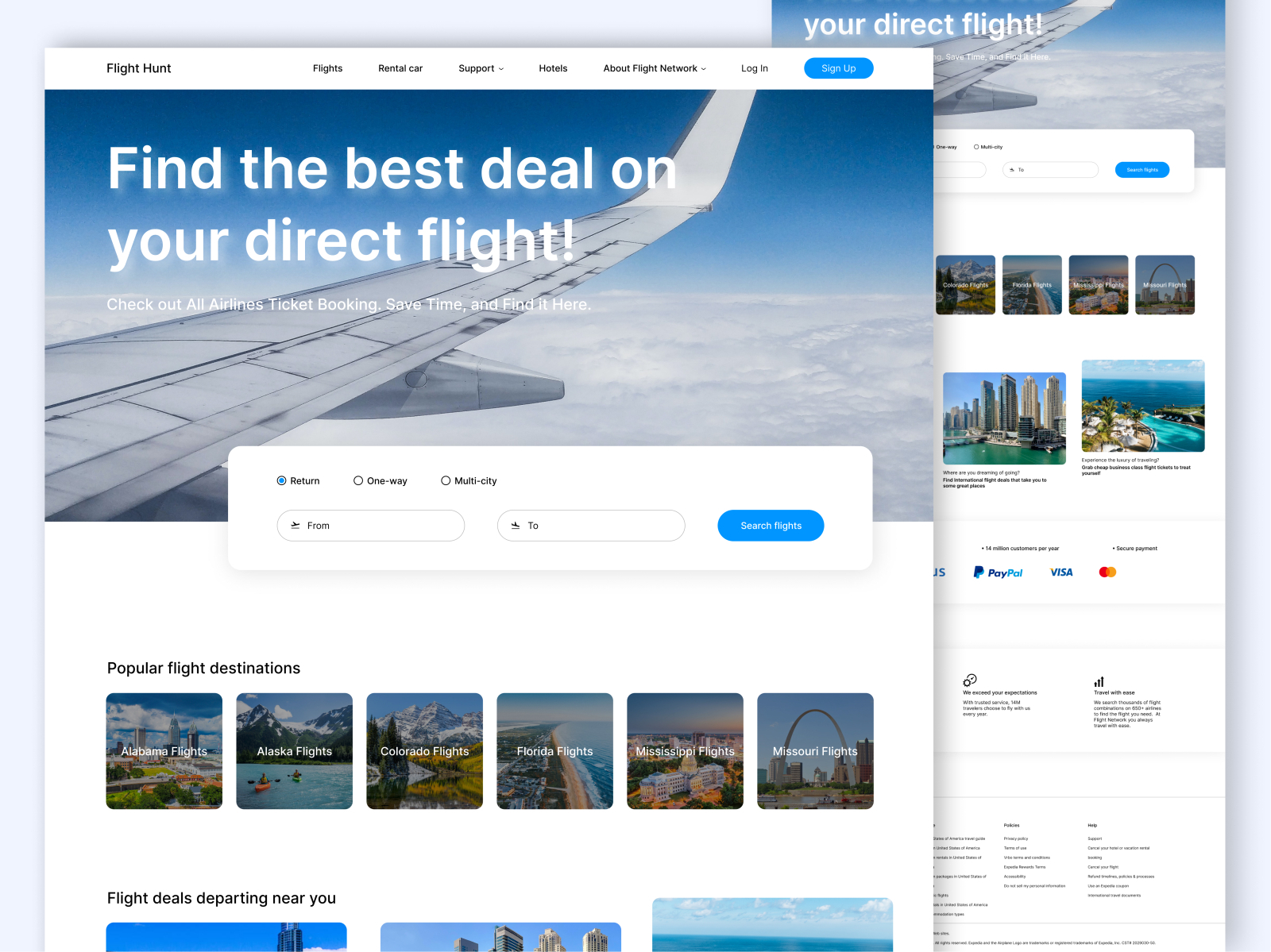The image is a screen capture of a web page showing two web page frames. The prominent frame in the foreground, positioned to the left, is a large square-shaped window. Within this frame, there is a photograph capturing the right wing and wingtip of an airplane in flight. The wingtip is set against a backdrop of a blue sky adorned with white clouds. Across the image, white text states, "Find the best deal on your direct flight." 

Below this text, three radio buttons are visible on a white background. The first button, labeled "return," is highlighted with a blue dot within the circle, indicating it is selected. Next to it are the options "one-way" and "multi-city." To the bottom right of these buttons, there is a blue "search flights" button. Beneath this section, various images and pictures of popular flight destinations are displayed.